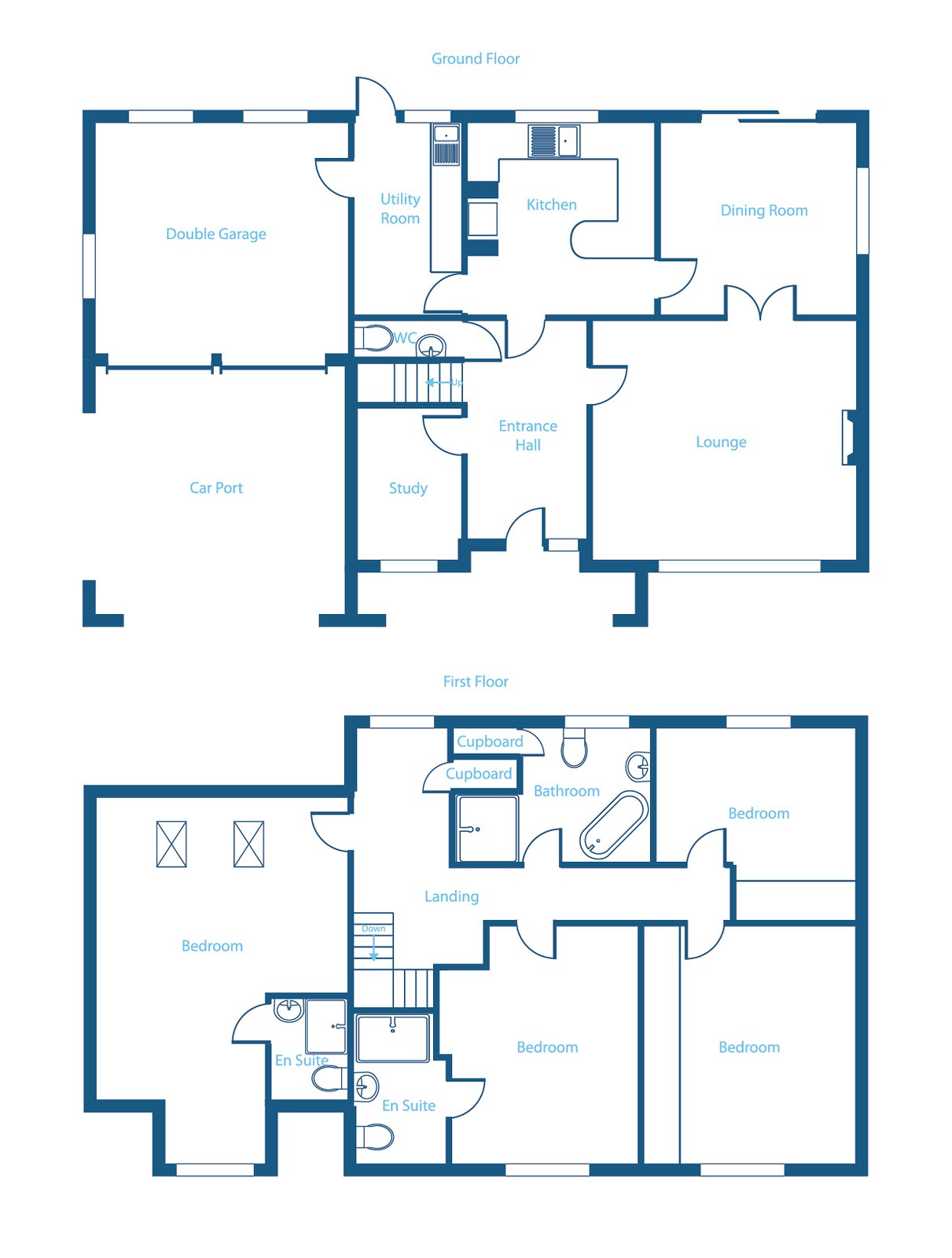This detailed computer-drafted floor plan features a rectangular house layout on a white background with precise blue lines delineating the structure. The ground floor includes a carport and a spacious double garage, accompanied by a utility room, kitchen, dining room, washroom, study, entrance hall, and lounge. Moving to the first floor, the layout reveals two bedrooms each with en-suite bathrooms, as well as two additional bedrooms sharing a separate bathroom located near the smaller bedroom at the top of the image. The plan also highlights the landing area and the stairway descending to the ground floor. The text and labels on the floor plan are clearly typed and highly legible, reflecting the meticulous nature of the digital drafting process. Overall, it provides a comprehensive and easy-to-read blueprint of the house's layout.